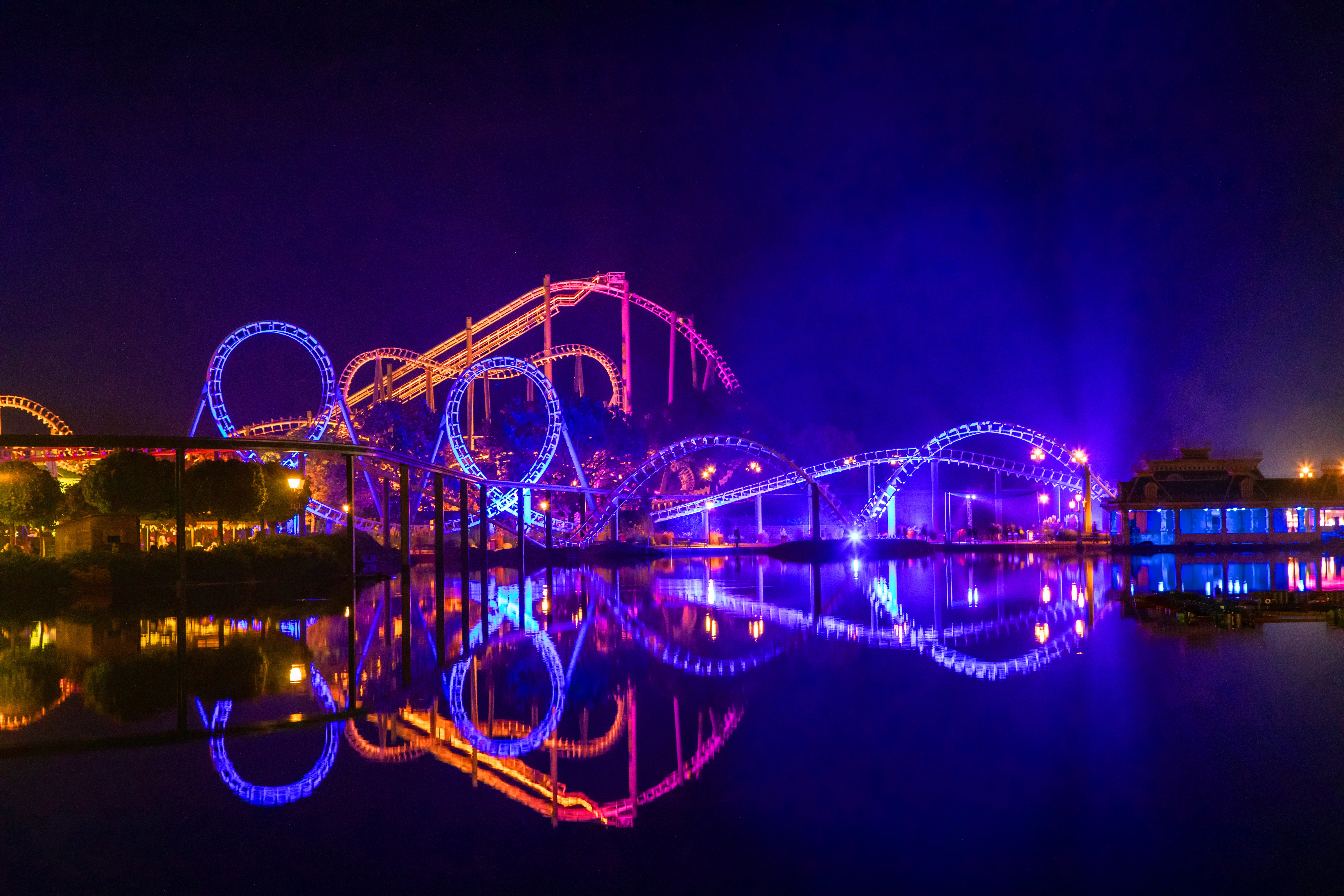This photograph captures a vibrant nighttime scene at an amusement park, with a central focus on a brightly lit roller coaster situated behind a dark, still lake. The roller coaster tracks are illuminated with an array of LED lights in colors ranging from pink and purple to orange and blue, casting vivid reflections on the water’s surface. The sky is completely black, framing the scene with a deep contrast, and the water appears dark and impenetrable. To the left, a warmly lit building with yellow LEDs and nearby green trees adds to the festive atmosphere. On the right side of the image, a boat adorned with blue LEDs mirrors its lights on the lake, enhancing the overall reflective effect. The amusement park's additional attractions, such as a pavilion and a boardwalk lined with shops, further contribute to the picturesque and lively setting. The colorful lights and their reflections create an enchanting extension of the structures onto the water, merging reality with its mirrored counterpart in a dazzling display.